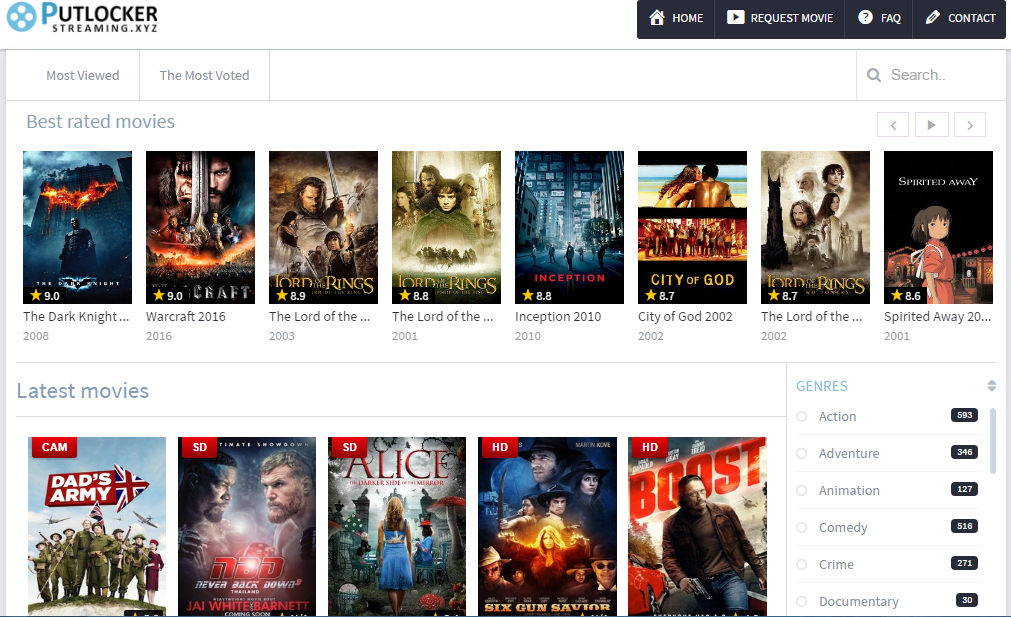Screenshot of the PotlockerStreaming.xyz website interface featuring four primary sections on the top right: Home, Request Movie, FAQ (Frequently Asked Questions), and Contact. Just below these, two links labeled 'Most Viewed' and 'Most Voted' are visible, alongside an empty search box positioned to the right. Beneath this navigation area is a section titled 'Best Rated Movies,' showcasing a horizontal list of films: "The Dark Knight" (2008), "Warcraft" (2016), "The Lord of the Rings: The Return of the King" (2003), "The Lord of the Rings: The Fellowship of the Ring" (2001), "Inception" (2010), "City of God" (2002), "The Lord of the Rings: The Two Towers" (2002), and "Spirited Away" (2001). Further down, a bold heading reads 'Latest Movies,' listing, from left to right, "Dad's Army," "Never Back Down," "Alice," "The Dark Side of the Mirror," "Six Gun Savior," and "Boost." At the bottom right of the page, a genre section displays various movie categories with their respective counts: Action (593), Adventure (346), Animation (127), Comedy (516), Crime (271), and Documentary (30).